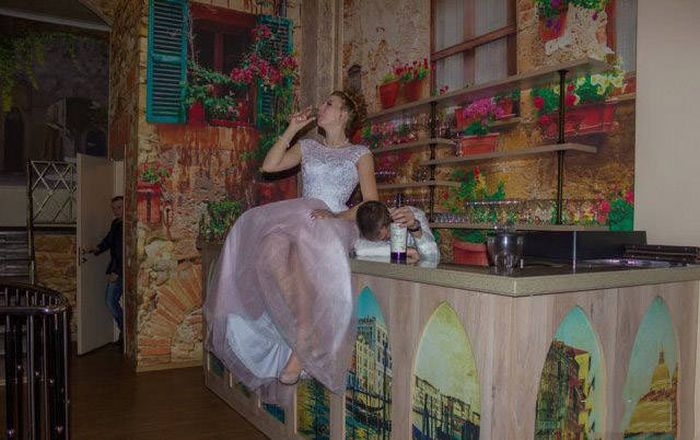In a rustic, Tuscan-styled bar with pastel pink hues, a woman in a pink and white dress reminiscent of Cinderella or a bridesmaid's gown is the focal point. The dress has a ballet pink, sheer skirt and a glittery white bodice, with her hair elegantly done up. She sits atop the bar, sipping a glass of what appears to be alcohol. The bar itself is painted to mimic shelves adorned with flowers, providing a charming facade. Behind the bar, a bartender in a white shirt appears to be asleep with his head in his hand, resting on a drink with a purple bottom. The backdrop features a typical bar setup with an array of glasses. To the right, a man in jeans and a black shirt enters the bar area through a door matching the bar's pastel pink color. The overall atmosphere hints at nighttime, reflected by the dim lighting and a dark window in the background.